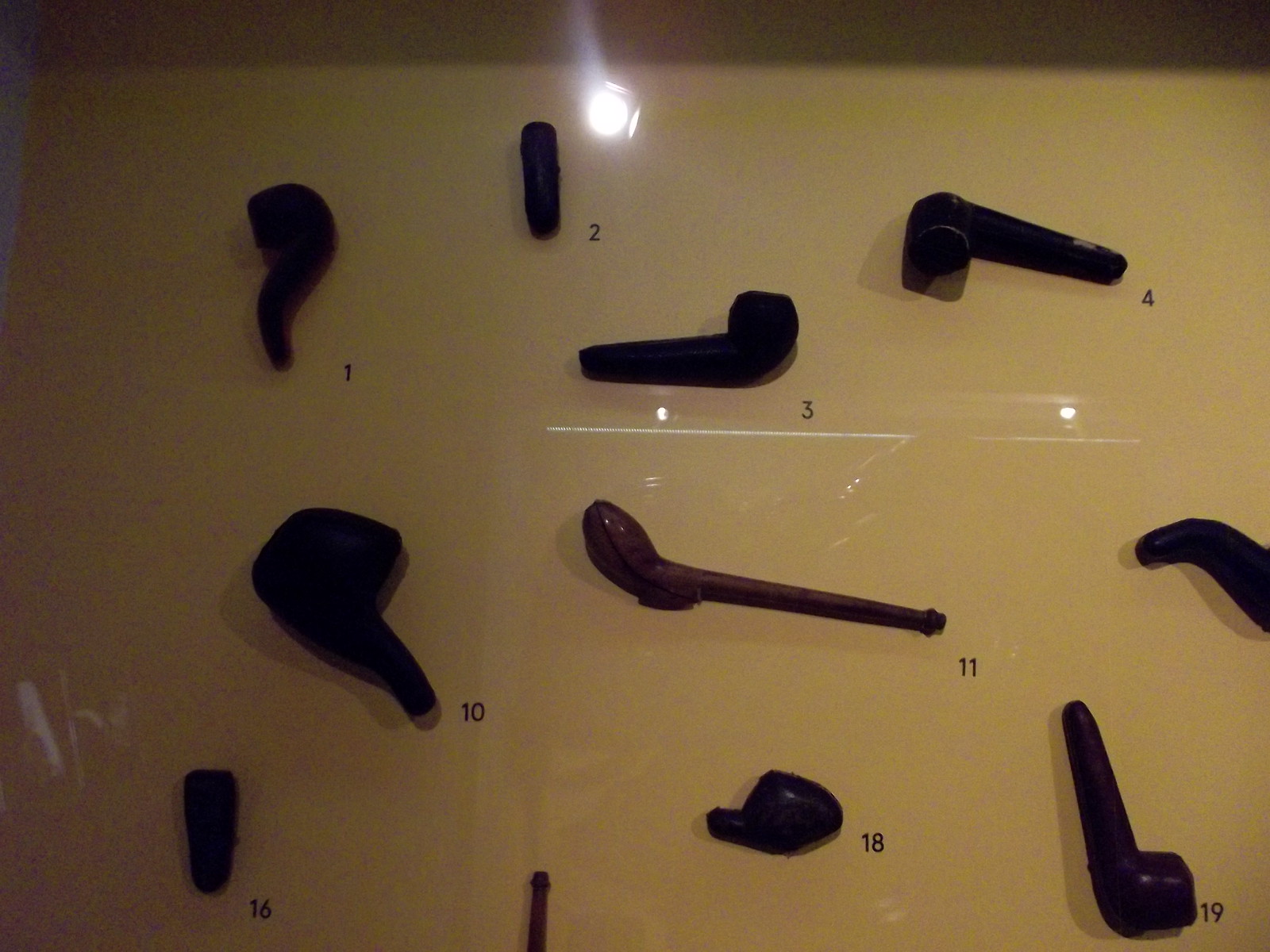The image is a realistic horizontal photograph taken through glass, evidenced by the visible reflections of lights and the camera flash. The background is predominantly white, possibly off-white due to poor lighting. Displayed on this white wall or tile are several smoking pipes, numbering around 9 to 11, all of which are varied in size, shape, and color (primarily brown or black). They are arranged in rows: the top row consists of four pipes labeled 1, 2, 3, and 4 in black text. Below, other pipes are labeled with numbers such as 10, 11, 16, 18, and 19, though some pipes and numbers, like 17, are partially visible. Each pipe has a distinct stem and bowl design, contributing to the display's eclectic aesthetic within the glass case.